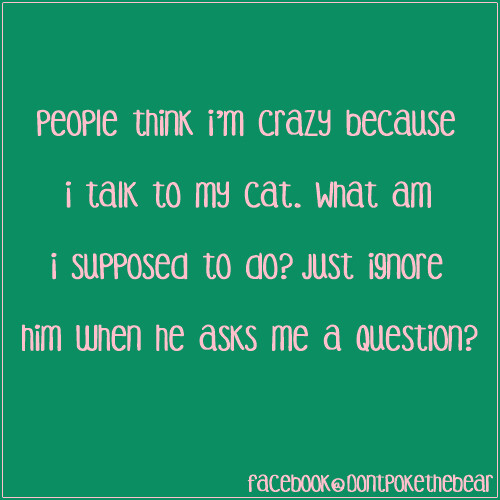This meme-style image features a medium green background with light pink text, creating a playful contrast. The text, written in a cartoonish font, reads, "People think I'm crazy because I talk to my cat. What am I supposed to do? Just ignore him when he asks me a question?" Positioned towards the center of the graphic, the text takes up most of the width and is vertically aligned for optimal readability. A subtle, one-pixel wide light pink border frames the image. In the lower right corner, there's a credit line indicating the source, which reads "Facebook at don't poke the bear," suggesting it was originally posted on Facebook by the page ‘Don’t Poke the Bear.’